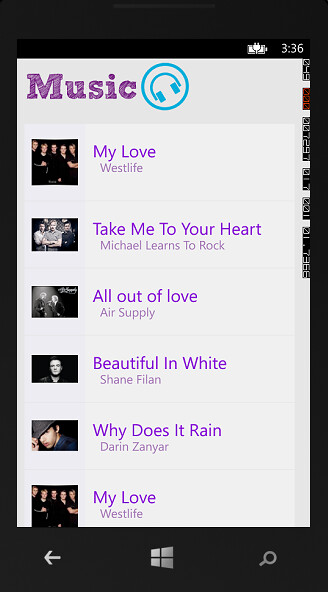The image is a screenshot of a mobile device, likely a Microsoft Windows phone, displaying a music app on its Browse page. The screen is predominantly framed in black borders. At the top-right corner, the battery icon is visible along with a plug-in symbol, and the time is shown as 3:36. Below this, the word "Music" is displayed in purple accompanied by a blue headphone icon.

The app features a list of songs, each accompanied by an artist's photo on the left side. The tracklist starts with "My Love" by Westlife, with the group's picture displayed next to it. Following are "Take Me to Your Heart" by Michael Learns to Rock, "All Out of Love" by Air Supply, "Beautiful in White" by Shane Filan, "Why Does It Rain" by Darren Zanier, and concluding with "My Love" by Westlife again.

At the bottom of the screen, on the left corner, there is a back arrow icon; the Windows logo is centered; and on the right corner is a search icon, indicating additional navigation options within the app.